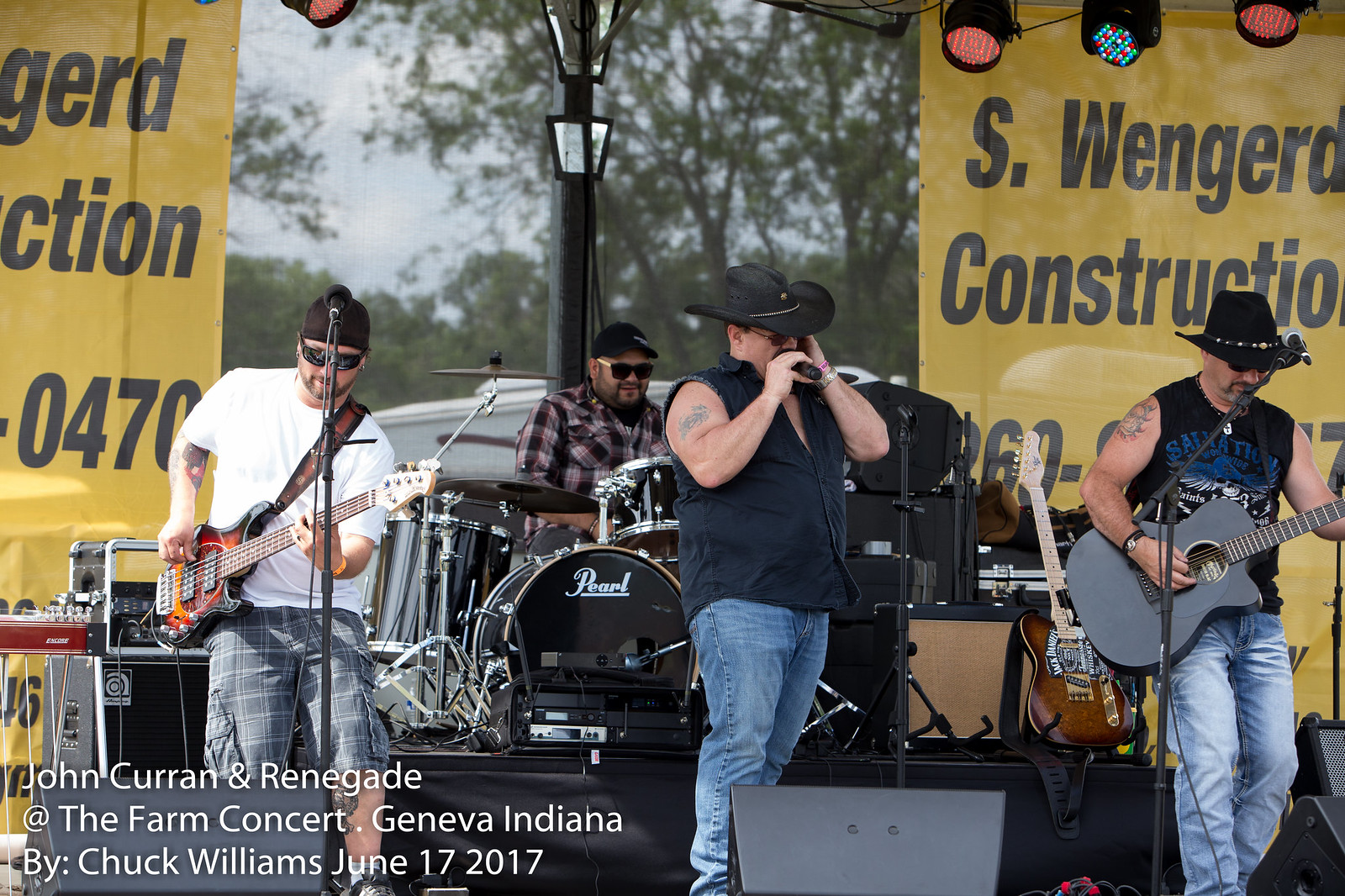This detailed caption for the poster photo of a band incorporates shared and specific elements from both descriptions:

The poster photo showcases a live performance by the band "John Curran and Renegade" at the Farm Concert in Geneva, Indiana, on June 17th, 2017, photographed by Chuck Williams. In the background, a drummer donning a black baseball hat and dark glasses is immersed in playing a black drum set. Center stage, the lead singer, wearing a black cowboy hat with a gold chain around it, holds a wireless microphone, dressed in a short-sleeved dark shirt and faded blue jeans. To the right bottom area, a guitarist is seen playing a gray-faced guitar, sporting a sleeveless black shirt with writing and symbols, showcasing tattoos on his upper arm, and wearing blue jeans. On the left, another guitarist in a white t-shirt and blue shorts down to his knees plays an electric guitar. Banners in the background hint at a construction advertiser, while the bottom left corner features white lettering with the event's name and details.